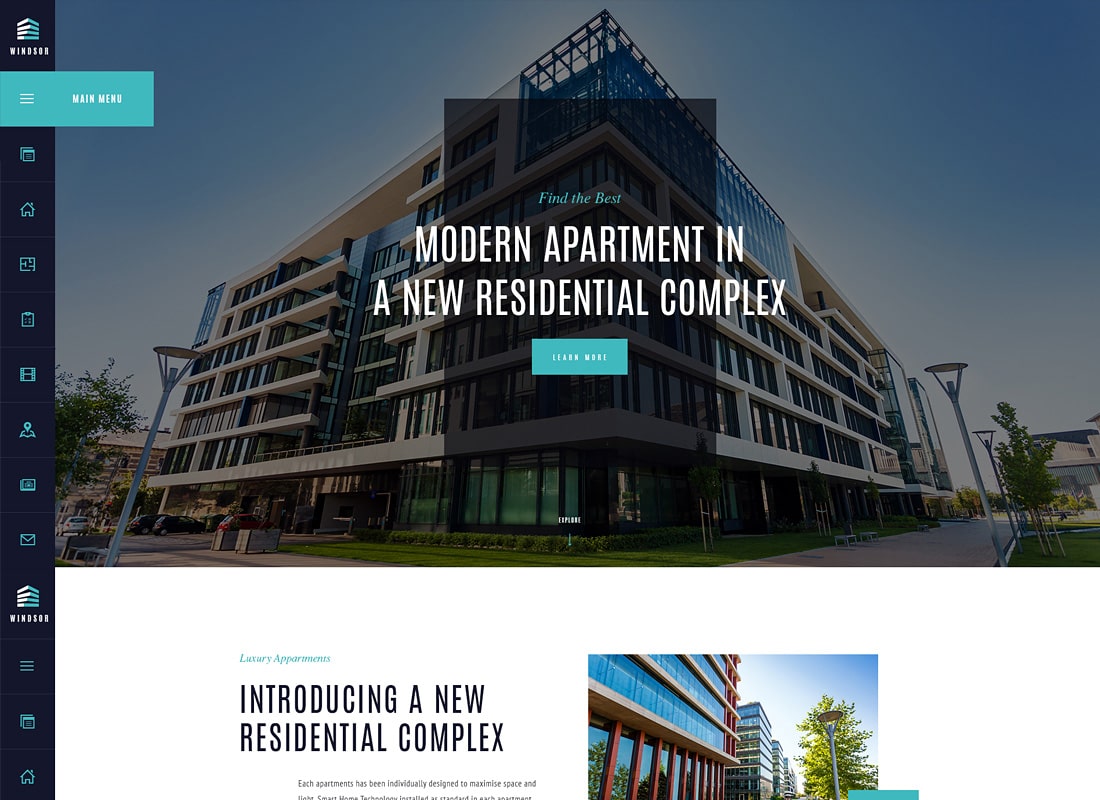The screen displays a website or digital brochure, potentially an application, for a property developer promoting modern apartments and a new residential complex. The background is dominated by an image of a sleek, contemporary building. Overlaying this background, in smaller green text,  are the words "Find the Best." In large, bold letters, it reads "Modern Apartment and New Residential Complex." Below this headline is a green "Learn More" button.

The page suggests that users can either buy or rent the apartments, though this is unclear. The lower part of the page mentions the introduction of a new residential complex, but it's partially cut off, indicating the need to scroll.

Along the left side, there is a vertical navigation bar with icons. At the top is a logo for the property company, possibly named Windrush or Windsor, and below it, a green box with the main menu icon. Additional icons appear beneath: a calendar, home, floor plans, a clipboard, film (which might indicate a virtual tour), a map, and some other icons that are partially obscured. Notably, the home icon appears twice, which may cause some confusion.

A smaller image of another modern apartment building framed by blue skies and a green tree is visible below the main image.